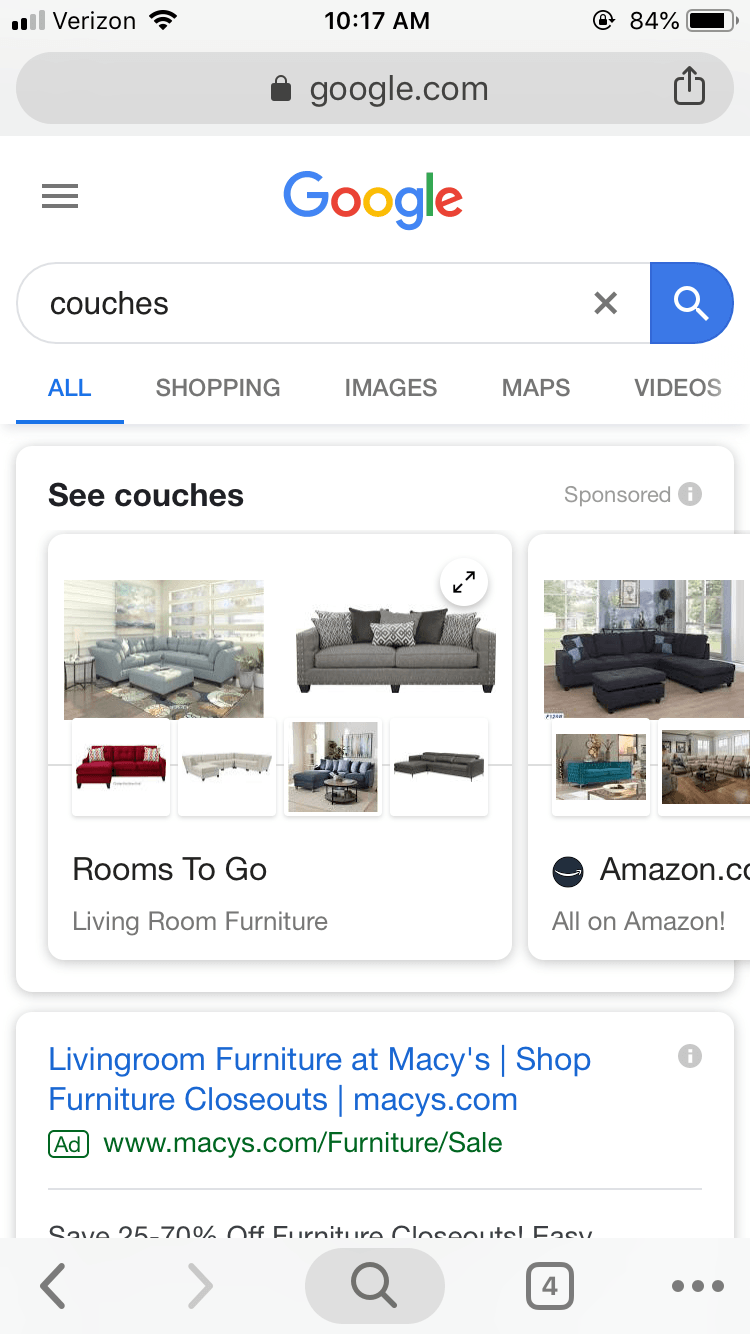The image showcases a Google search screen on a Verizon cell phone, taken at 10:17 a.m. with the battery at 84%. In the Google search bar, the user has typed the word "couches," and beside it, there's an 'X' to clear the search, followed by a blue button featuring a magnifying glass icon. Below the search bar, search results display, starting with ads for "Rooms To Go" and "Amazon.com."

Further down, the first search result in blue font reads "Living Room Furniture at Macy's," with a sub-link to shop closeouts at Macy's (www.Macy's.com/furniture/sale). Scrolling through the search results, there are images of various couches: some presented in an isolated view without any background, and others depicted within home settings, providing context on how they would look in a furnished space. The image section shows multiple listings, with one grouping containing six couch images and another group displaying three, with part of the set cut off from the screen capture.